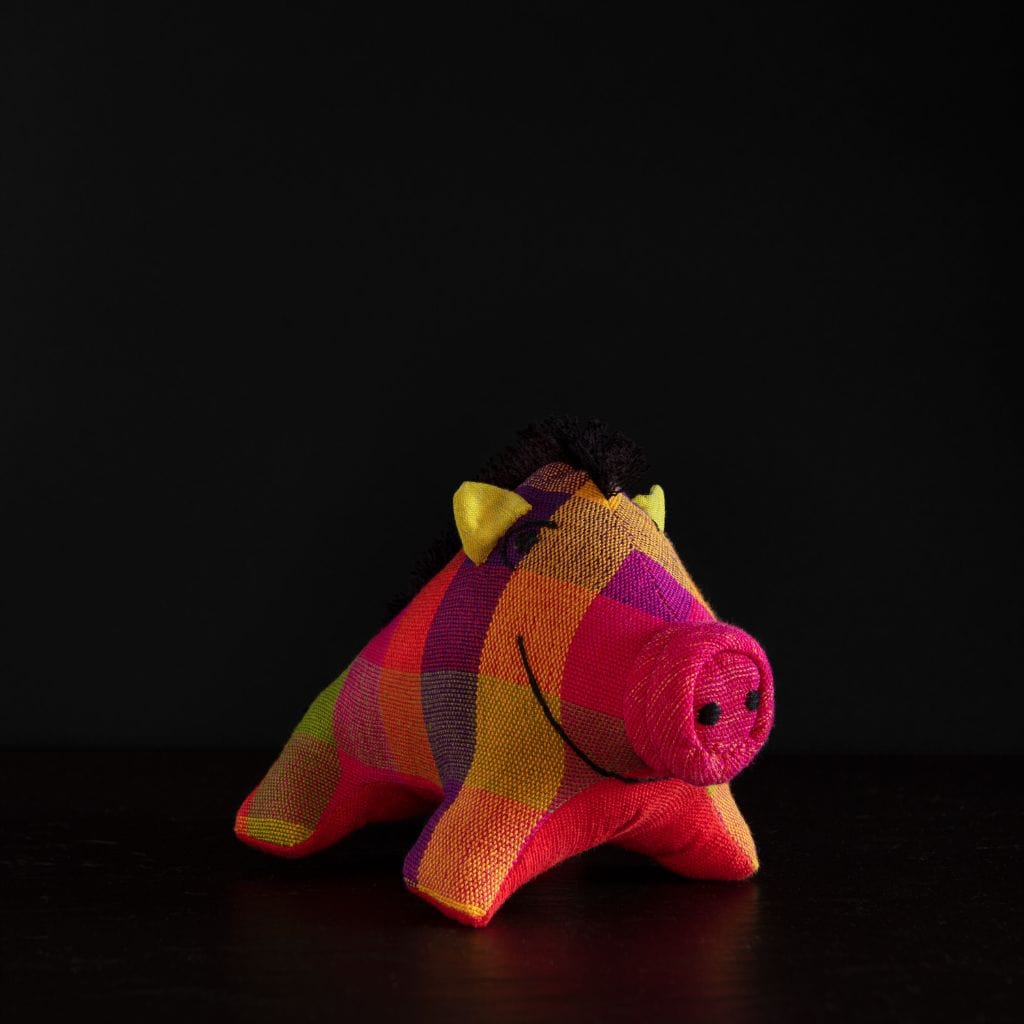Against a jet-black background, a distinctive hand-sewn stuffed pig takes center stage. Its body is crafted from a vibrant plaid fabric featuring squares in yellow, purple, blue, green, and orange. This whimsical pig has bright yellow, fabric ears that stand straight up, adding to its playful appearance. The pig's face is adorned with large, cartoonish black eyes, and a cheerful black yarn-stitched smile that brings it to life. A prominent double-layered pink snout sits at the forefront, complete with two black stitched nostrils. Atop its head, a strip of black fabric mimics a fuzzy mohawk, lending it a quirky, charming personality. The pig's four legs are visible, suggesting it's standing proudly, showcasing the handiwork of its creator. The plush texture and colorful patchwork make this little pig an endearing piece of art.